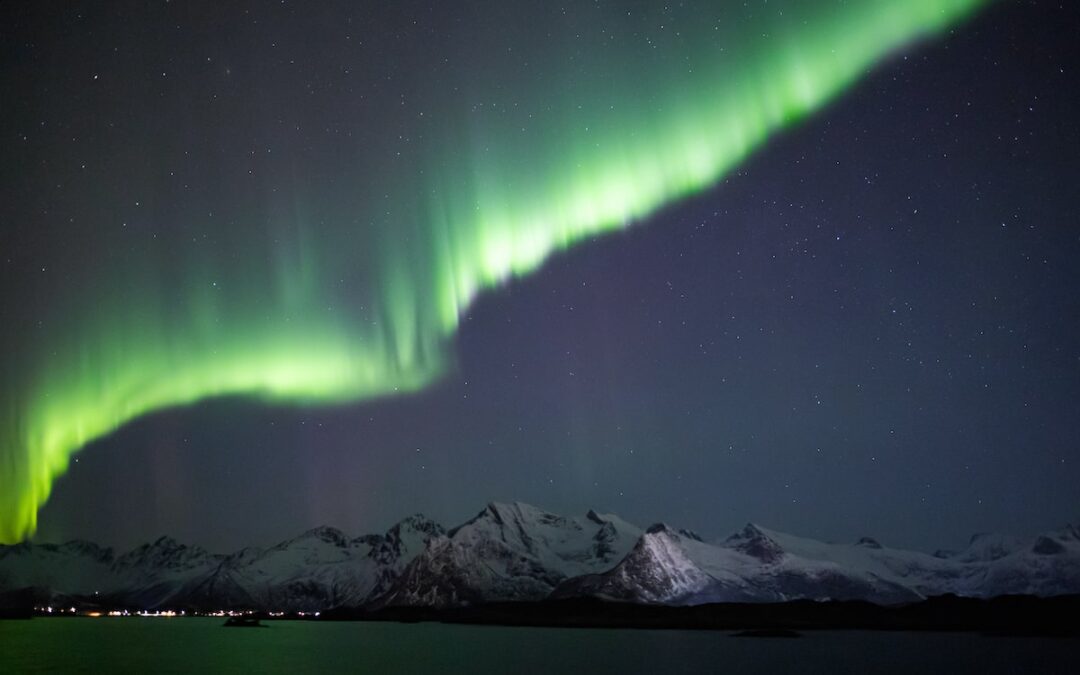This breathtaking photograph captures the ethereal beauty of the Aurora Borealis illuminating a mountainous landscape. Dominating the night sky, the vibrant, yellow-green aurora extends diagonally from the bottom left to the top right of the image, with bright light and radiating extensions giving an ethereal feel as if descending from the heavens. Below this celestial display, the rugged mountain range spans the entire width of the photo, its dark contours subtly accented with shades of black, blue, and hints of purple. Highlighting the peaks, the aurora adds a mystical glow to the snow-dappled summits, especially noticeable towards the center. In the bottom left corner, a string of tiny lights, possibly from boats or a distant city, flickers just above the vast water that stretches towards the mountain base. The star-speckled night sky frames this stunning natural phenomenon, blending seamlessly with the luminous green light of the aurora, together creating a dazzling spectacle.